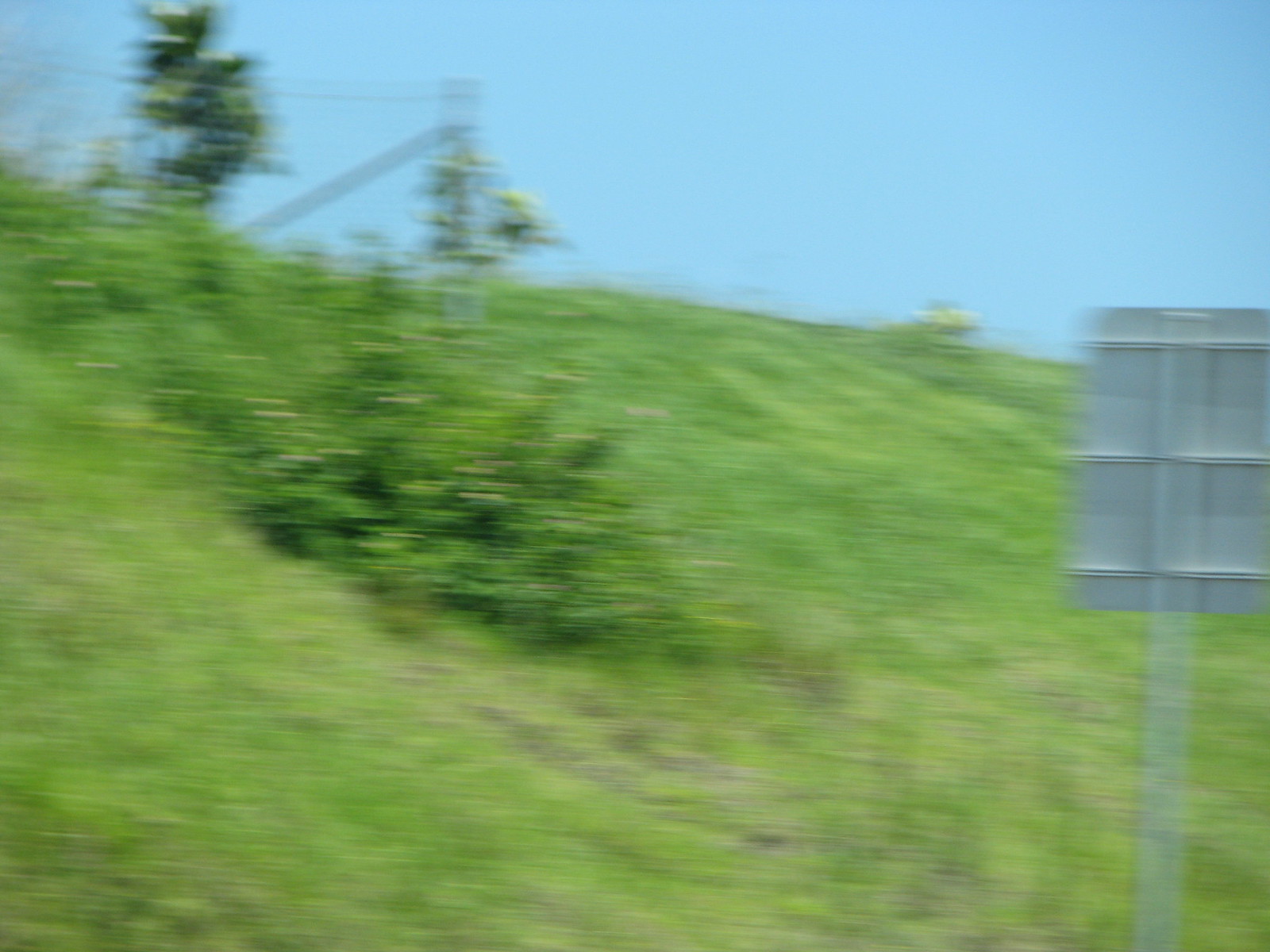**Caption:**

This image, despite its blurriness, captures a scene dominated by a vibrant blue sky stretching across the entire top portion. Towards the upper left, a structure is partially visible, though indistinct, adding a mysterious architectural element. Closer to the top left corner, the outline of a green tree can be discerned, its foliage blending into the skyline. The lower two-thirds of the photo are predominantly green, indicating a grassy area. Left of center, a darker green patch stands out, possibly a large bush. On the far right, the back of a street sign is visible, adding an urban touch to the natural elements of the scene.